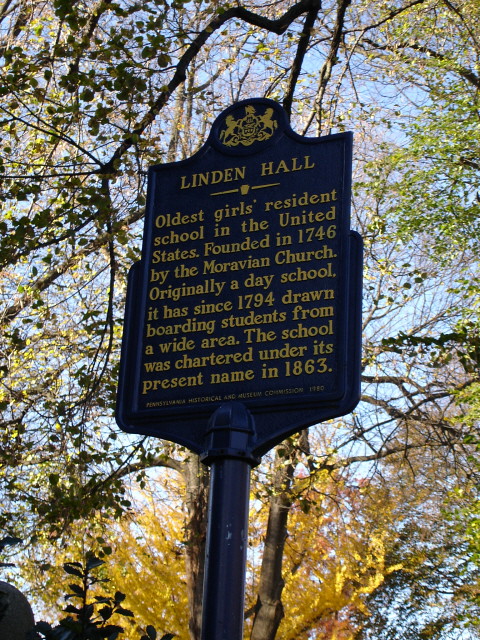The image showcases an informational signboard for Linden Hall, the oldest girls' residence school in the United States. Situated under a canopy of tree limbs adorned with green and yellow leaves, the picture is taken from a low angle looking upward. The background sky appears to be a clear blue, possibly with a white cloud hovering. The signboard, mounted on a creatively designed blue pole, displays text in golden yellow. At the top of the sign, a logo featuring two horses flanking an indiscernible design is prominent. Below the logo, the heading "Linden Hall" is underlined, followed by detailed historical information: "Oldest Girls' Residence School in the United States. Founded in 1746 by the Moravian Church. Originally a day school, it has since 1794 drawn boarding students from a wide area. The school was chartered under its present name in 1863." At the bottom, a small footnote reads, "Pennsylvania Historical and Museum Commission, 1880," although the year is not very clear.